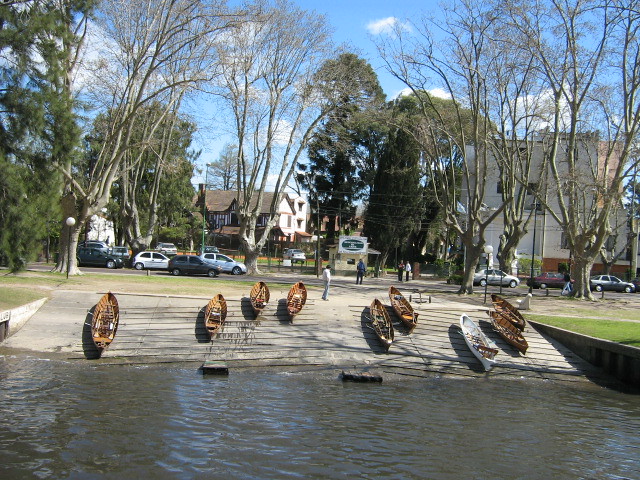The photograph captures an outdoor scene set in what appears to be a small-town area by a pond or lake. The scene is dominated by a sloping concrete jetty leading into opaque, dark water with slight ripples. On the jetty, there are nine wooden canoes—eight of them brown and one white—carefully arranged and facing towards the water. At the top of the jetty stands a person dressed in white, their face not visible. Surrounding the water, the lush greenery of large trees and well-manicured lawns add a serene touch, while scattered buildings and parked cars point to a suburban setting. The scene features pathways and small streetlights, adding to the quaint, small-town vibe. In the background, there are two-story houses and a sign written in white and green, enhancing the picturesque yet tranquil ambiance of the whole setting.